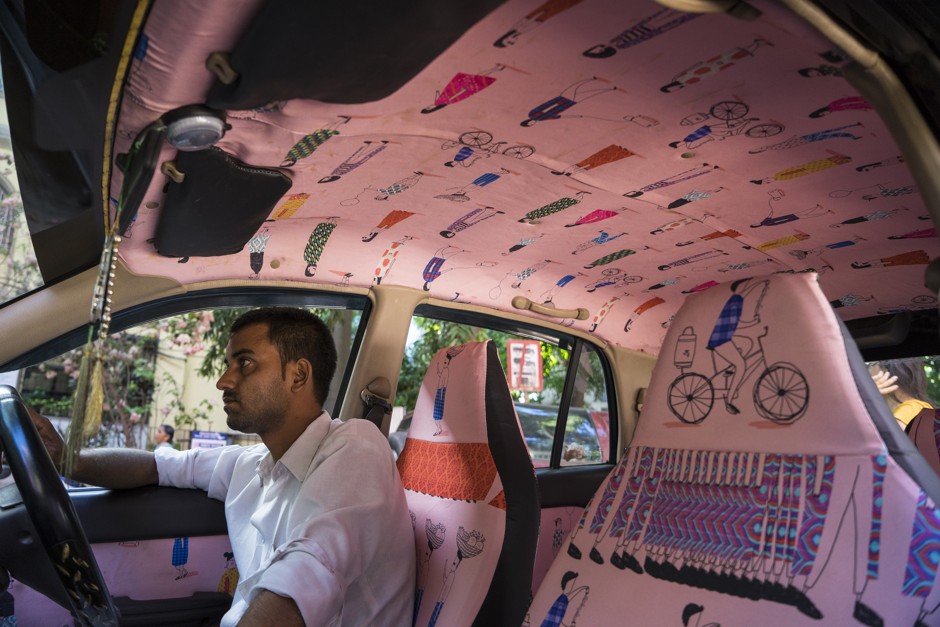The image depicts the interior of a van being driven by a man on the right-hand side, indicating that the location is likely outside of the United States. The man has short, dark hair and is wearing a white, long-sleeve button-down shirt with the sleeves rolled up. He has his right arm resting on the window's edge and his right hand on the upper right part of the black steering wheel. His left arm hangs down to his side.

The van’s interior is uniquely decorated with a vibrant, cartoonish design. The roof features a white or pink background adorned with colorful illustrations, including bicycles and various characters in bright outfits. These illustrations continue onto the seat covers, with the driver's seat displaying a light-colored background with an orange stripe and additional blue and multicolored images. The top of the passenger seat also showcases colorful vertical rows and images of people, contributing to the lively and whimsical decor.

Hanging from the rearview mirror are chains with tassels, adding to the eclectic aesthetic. Outside the windows, the scenery includes trees, people walking on the sidewalk, and a yellow building, indicating the van is driving through a neighborhood. The detailed drawings and unique character of the vehicle’s interior create a striking contrast to the mundane setting outside.